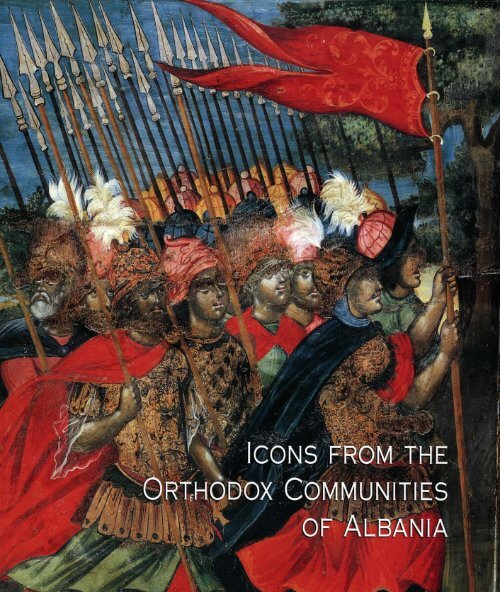The image portrays a detailed, vibrant painting reminiscent of ancient times in Albania, depicting an intense scene with soldiers. Centered is a large group of armored soldiers, all rushing towards the right, brandishing metal-tipped wooden spears that are oriented upwards into a bright blue sky. The soldiers are clad in an array of colored attire, primarily dominated by red capes, yellow and black headdresses, and some elements of green and gray. To the right, a prominent figure stands out, brandishing a red flag adorned with a gold tip, while this figure is distinctively dressed in a blue cape and a red skirt. The backdrop on the right features a tree with sparse leaves, adding depth and context to the scene. Overlaid at the bottom right in contrasting white text, the title "Icons from the Orthodox Communities of Albania" is prominently displayed, suggesting this may be cover art for a book. This composition collectively evokes the historical essence and cultural heritage of the region.